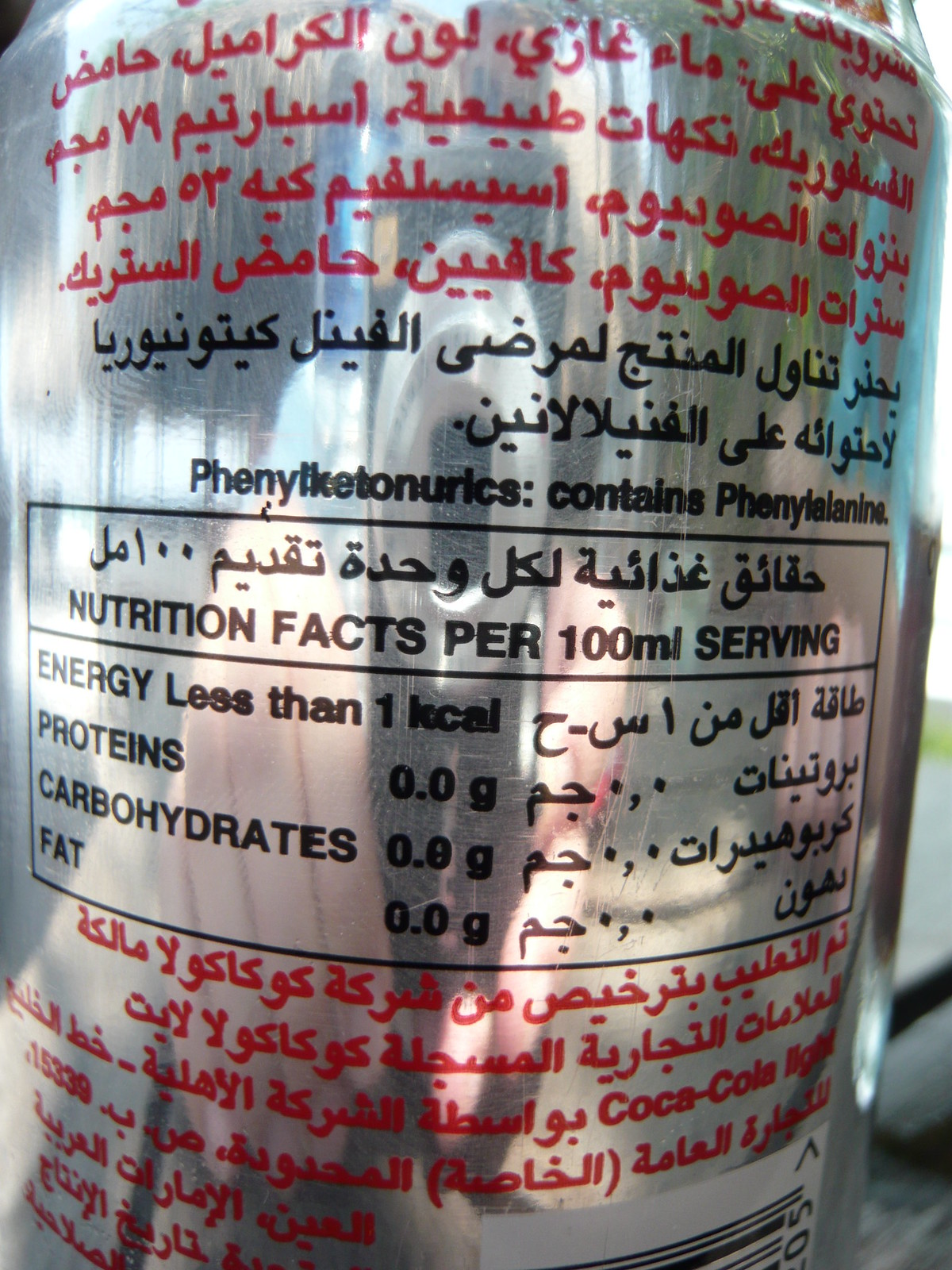This color photograph, slightly taller than it is wide, features a close-up shot of a shiny silver beverage can, occupying almost the entire frame. The can, made from a reflective metal, mirrors a partially visible cell phone and other indistinct shapes. Adorned with a mix of foreign and English text, the can’s design primarily consists of what appears to be Thai script in both red and black ink. English text is present in the form of a black-outlined square detailing nutritional facts per 100 milliliter servings. The lower part of the can returns to displaying red foreign characters, completing its intricate and multicultural labeling.